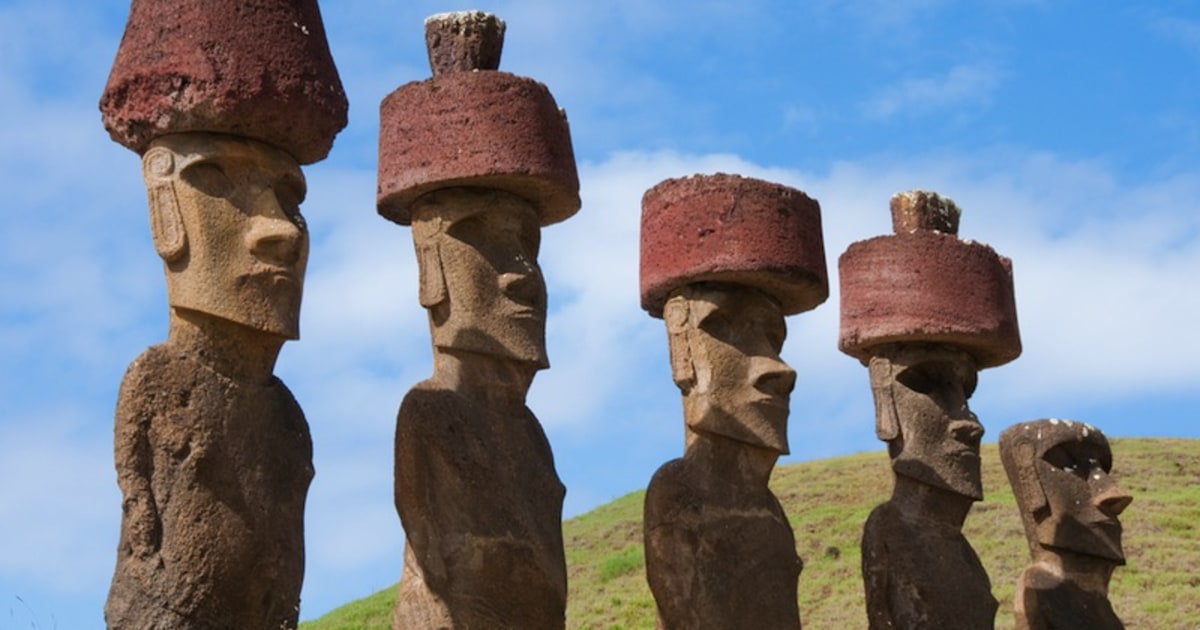The image features five stone-carved statues, reminiscent of Polynesian artistry, like those seen in Tahiti or Hawaii. Carved from lava rock, the statues have brown bodies with chiseled small, short arms, and short brown necks that transition to tan-colored faces. Their faces are characterized by flat features, prominent noses, square chins, and recessed eyes. The statues display ear flaps, some suggesting the presence of earrings. Crowning four of the five statues are red stone hats, with a couple featuring additional wooden top pieces, giving the appearance of helmets or toppers. One statue, however, lacks this head adornment entirely. The outdoor scene is set against a backdrop of blue skies with white puffy clouds, and a hill with low-growing grass and plant life, suggesting a locale akin to Easter Island in Chile, famous for such monumental statues.